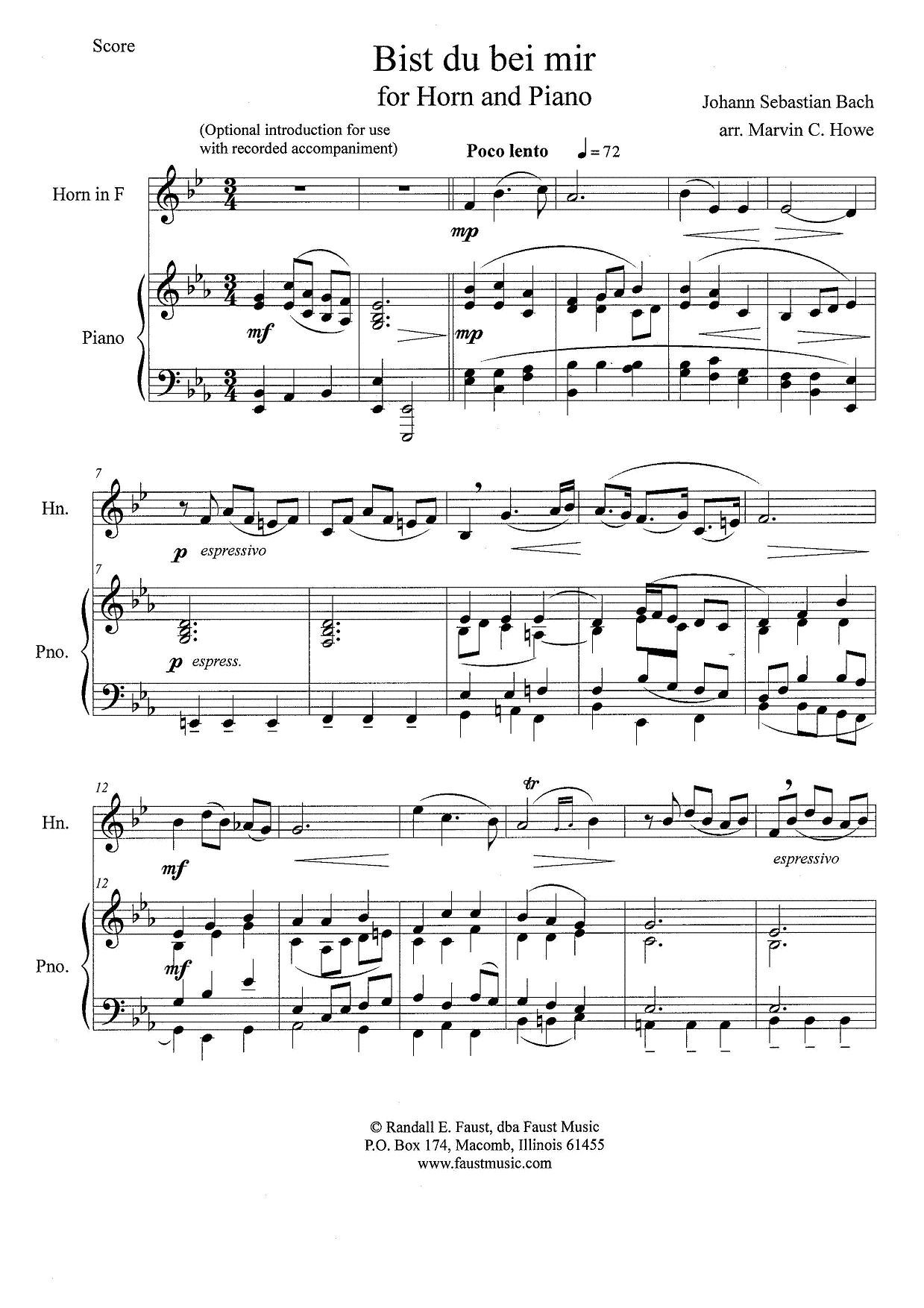This image shows a detailed page of sheet music titled "Bist Du Bei Mir" for horn in F and piano, originally composed by Johann Sebastian Bach and arranged by Marvin C. Howe. The music is intended also for optional use with recorded accompaniment. The top section of the page is designated for the horn in F, while the bottom sections are for piano, with three distinct rows of musical notation for both instruments. Notations include various musical expressions such as "MP," "P," "expressivo," and "MF." The background of the page is white with black musical notes and text. At the bottom right-hand corner, it indicates the copyright information: Randall E. Faust, Faust Music, P.O. Box 174, Macomb, Illinois 61455, along with the website www.faustmusic.com.